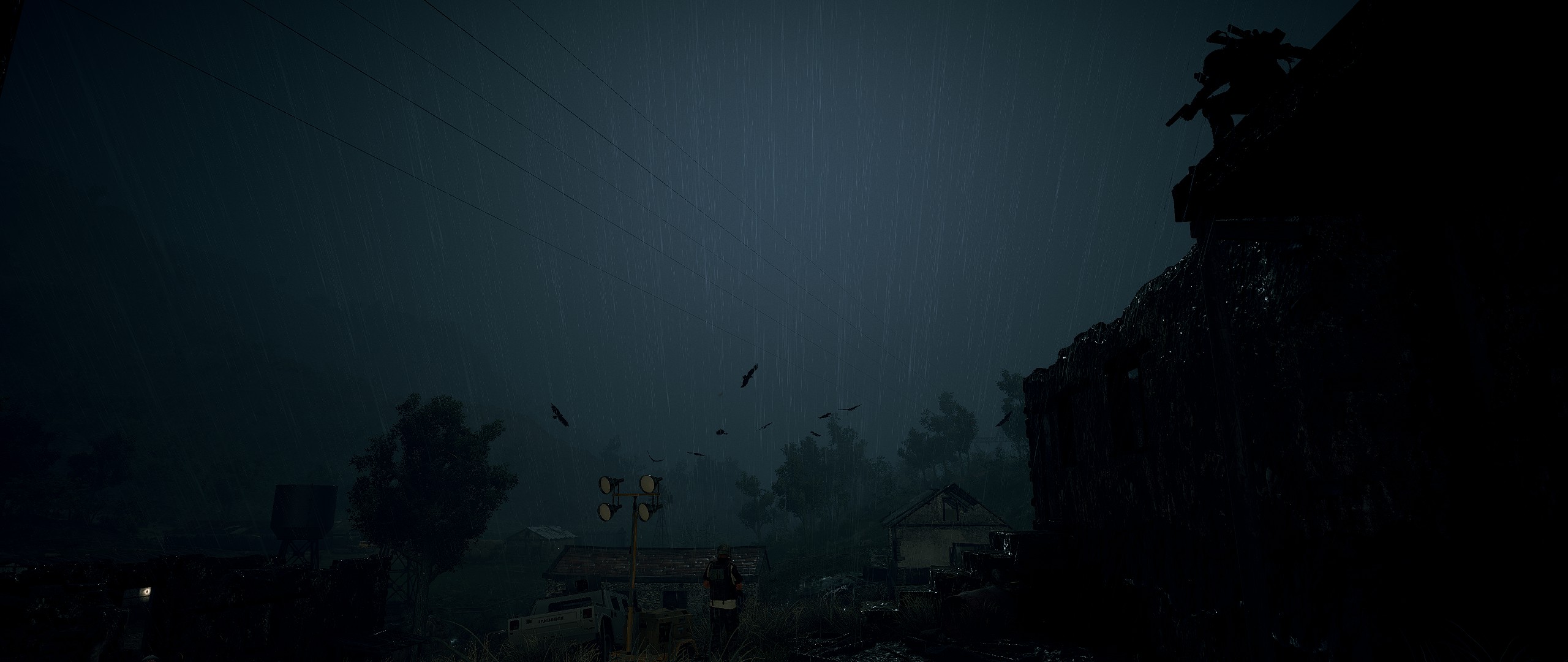This image, potentially a photograph or painting, depicts a very dark and stormy scene, possibly during a severe weather event such as a wildfire or tornado. The sky is an ominous gray-black, filled with swirling debris or birds, creating a sense of chaos. The right side features a dark, mountain-like silhouette, while a smaller building with a tan color and brown roof stands adjacent to it. Scattered across the scene are specks of light, possibly from windows of distant houses.

At the bottom center, a person is visible, seemingly walking away from the camera, adding an element of human presence to the otherwise desolate landscape. To the left of the person is a white, old-timey truck, parked with its bed towards the photographer. A tree next to the truck appears to be blowing in the wind, emphasizing the stormy conditions. 

A prominent light pole with four yellow lights stands towards the middle of the image, casting a faint glow amidst the darkness. Electrical wires stretch from the top left to the center, gradually disappearing into the mist. The entire scene is enveloped in a heavy, misty grayness, with windswept trees and a background shrouded in a murky haze, epitomizing the tumultuous nature of the depicted storm.